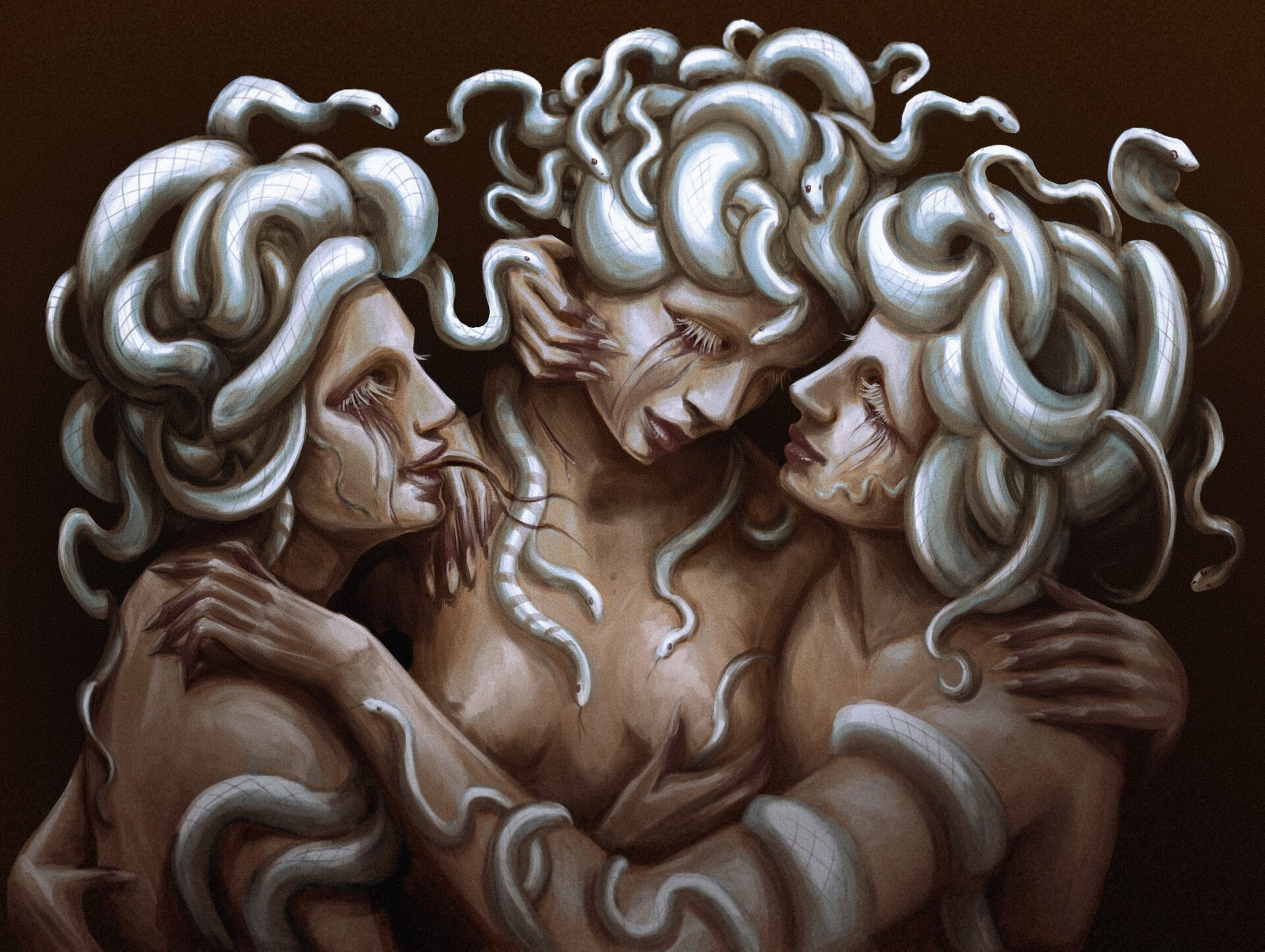The image is a contemporary painting, possibly computer-generated, depicting three naked gorgons, likely Medusa and her sisters from Greek mythology, all with serpents for hair. The central gorgon appears melancholic, her eyes slightly downcast and adorned with long eyelashes that touch her cheeks. She is being embraced on either side by the other two gorgons. The gorgon on the left is particularly striking with a snake-like forked tongue protruding from her mouth and similarly long eyelashes. She is clutching the breast of the central figure. The third gorgon on the right also has her arms intertwined around the central figure, completing the familial embrace. The serpents are not confined to their heads but coil around their necks and arms as well. The trio stands against a dark background, their expressions conveying a mixture of indifference and sorrow. The painting, detailed yet not overly intricate, exudes a compelling, dark atmosphere that captures the mythological essence of the gorgons.